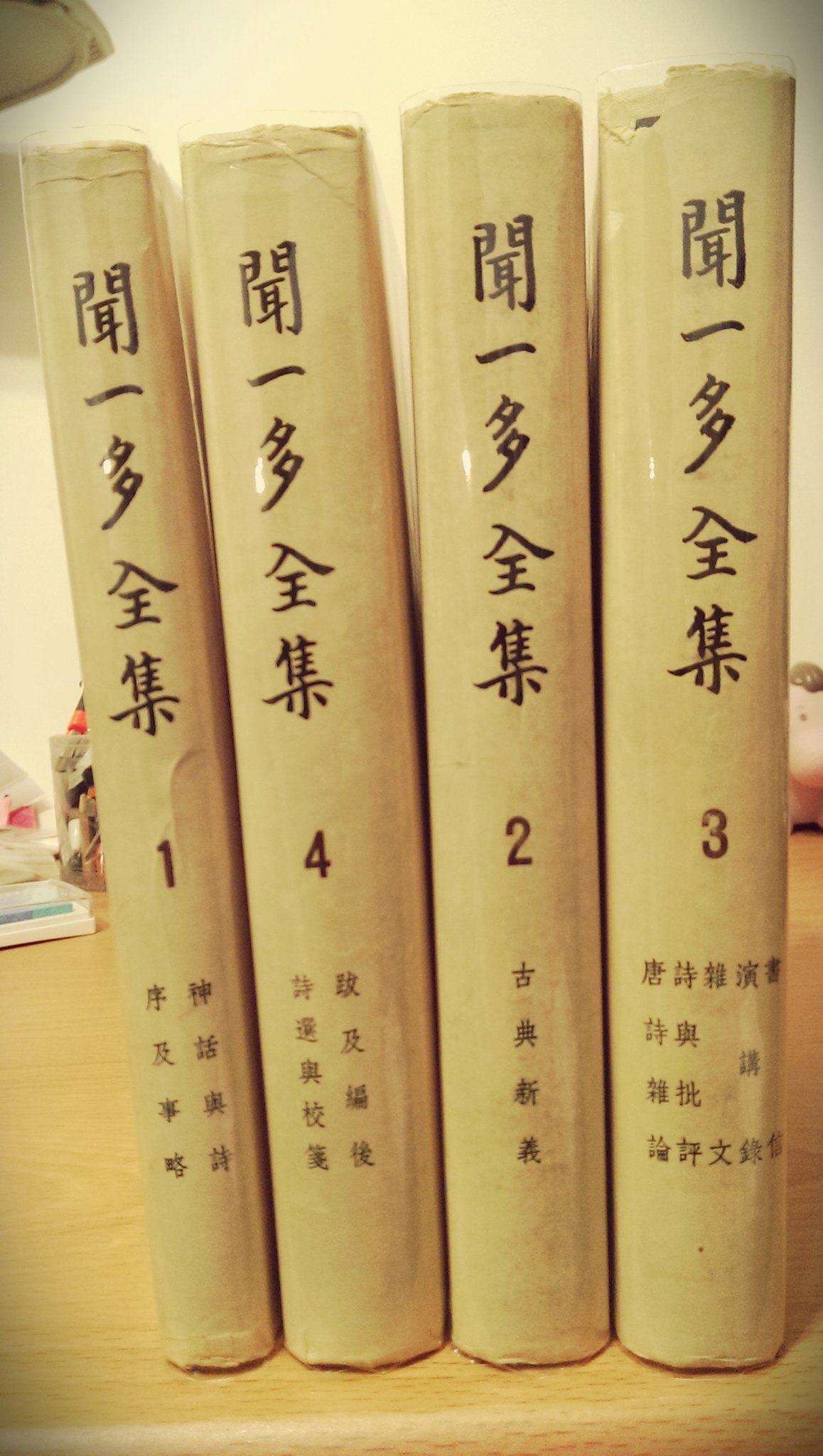This image showcases a close-up of four upright books standing on a light brown wooden surface, with a white wall in the background. The books feature a tan or beige hue and have black Japanese characters adorning their spines. Each spine prominently displays numbers in an unconventional sequence: one, four, two, and three. Below these numbers, smaller Japanese characters line the bottom portion of each spine. To the right side of the books in the background, partially cut off, is a small white plastic object with blue and teal buttons. Just barely visible is what seems to be a figurine or toy with a pink face, likely representing an animal such as a pig or hippopotamus, adorned with a round toupee and a small brown eye. This scene is well-lit, further highlighting the detailed elements.